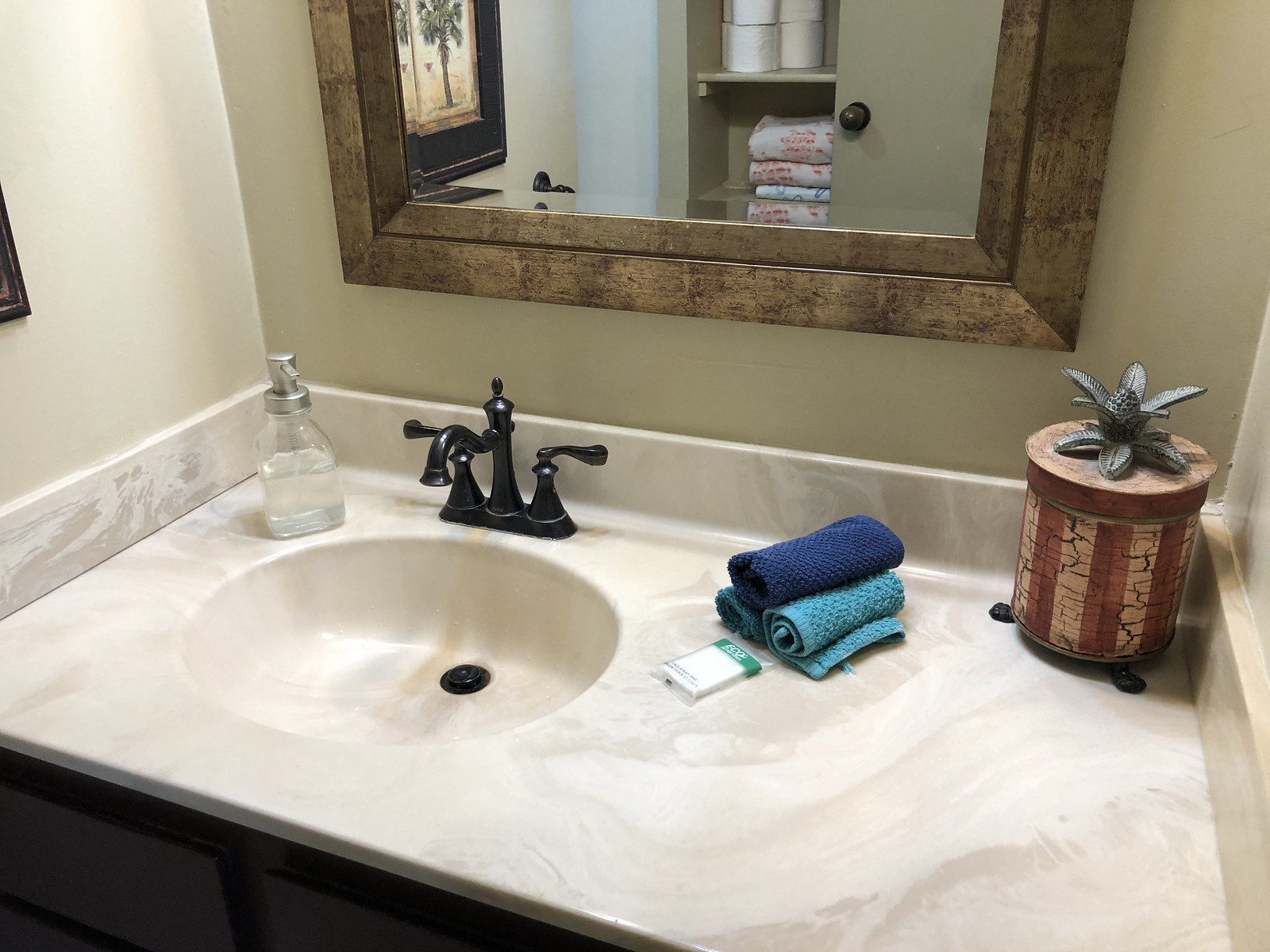The image captures a quaint and well-organized bathroom with a soothing, warm ambiance. The walls are painted in a tannish-yellowish hue, providing a cozy backdrop. Visible are the left, back, and right walls. The back wall is adorned with a centered mirror that reflects part of the bathroom door and a set of neatly arranged shelves behind it. The top shelf holds four neatly rolled toilet paper rolls, while the shelf below is stocked with pristine white towels, some featuring patterns of red and blue circles.

To the left of the shelves, a painting of a tree adds a touch of nature to the decor. Outside the mirror's reflection, a granite countertop spans part of the image, supported by dark brown drawers located in the bottom left corner. On the counter, three hand towels create a pyramid; the top towel is dark blue, and the two underneath are light blue. The sink, placed centrally on the countertop, boasts a faucet with a dark, possibly copper, handle and two knobs for adjusting hot and cold water. A small plant in the top right corner of the countertop adds a fresh, natural element to the bathroom.